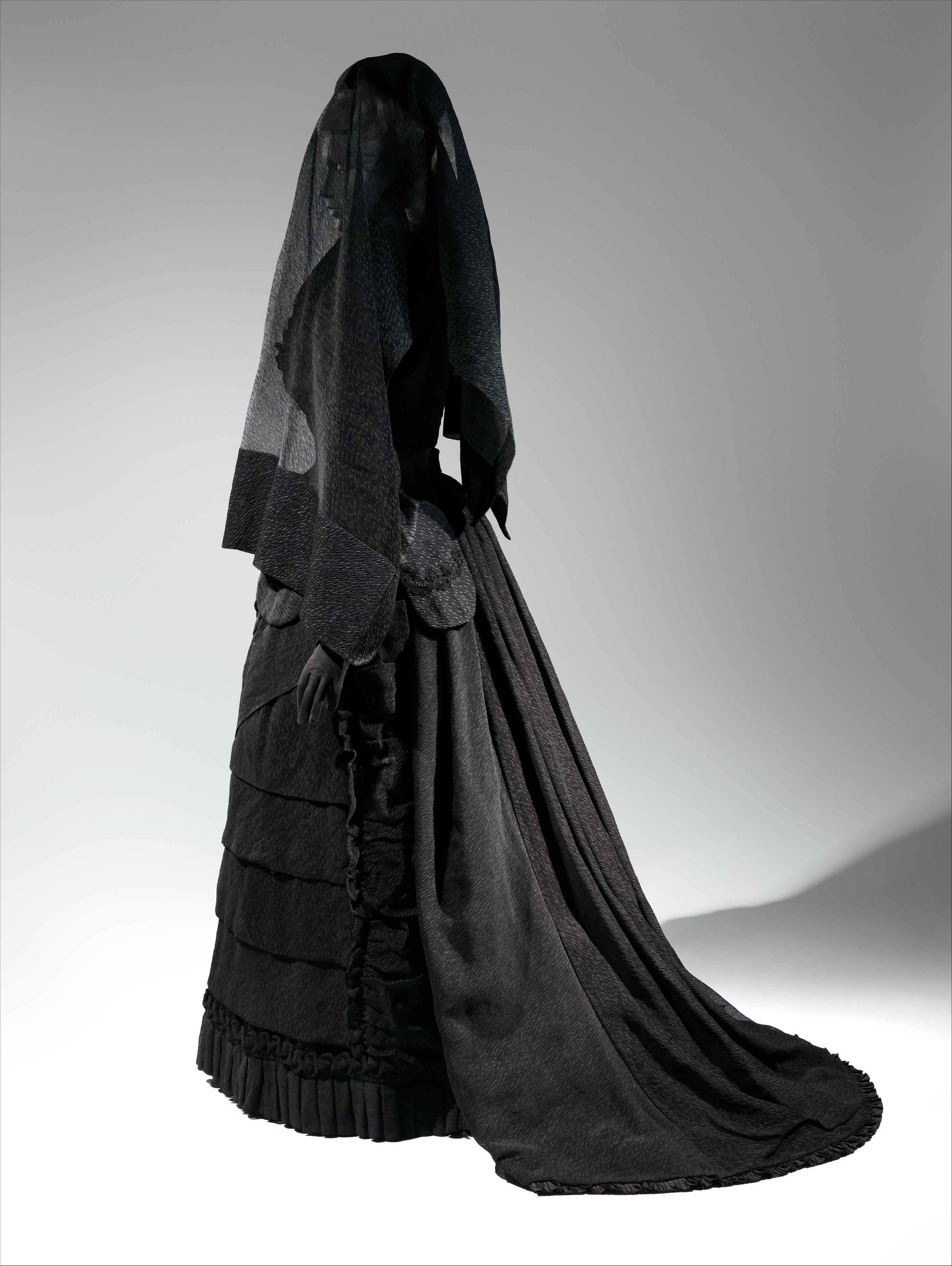This captivating photograph captures the side profile of a woman—or possibly a mannequin—draped in a striking all-black gown that exudes a gothic aesthetic. The dress, reminiscent of a wedding gown yet bathed in an entirely black hue, features a torso-hugging design that flares dramatically from the hips down into a long, flowing train of fabric. The front of the gown is adorned with pleated sheets and frilled edges, adding a layer of intricate detail to its stark elegance.

Her head is covered by a black veil that cascades down in a lacy pattern, transitioning from a transparent material at the top to a denser, opaque fabric towards the bottom. Though her face is partially obscured by the veil, the shadowy outline and faint features of a woman are discernible. Her eyes appear somewhat shadowed, adding to the mysterious aura.

She stands against a grey and white gradient background, where the light casts her shadow to the right, creating a unique pattern that complements the gothic theme of the attire. Her hand, visible and darkened to a charcoal hue, further contributes to the overall enigmatic and timeless quality of the image.